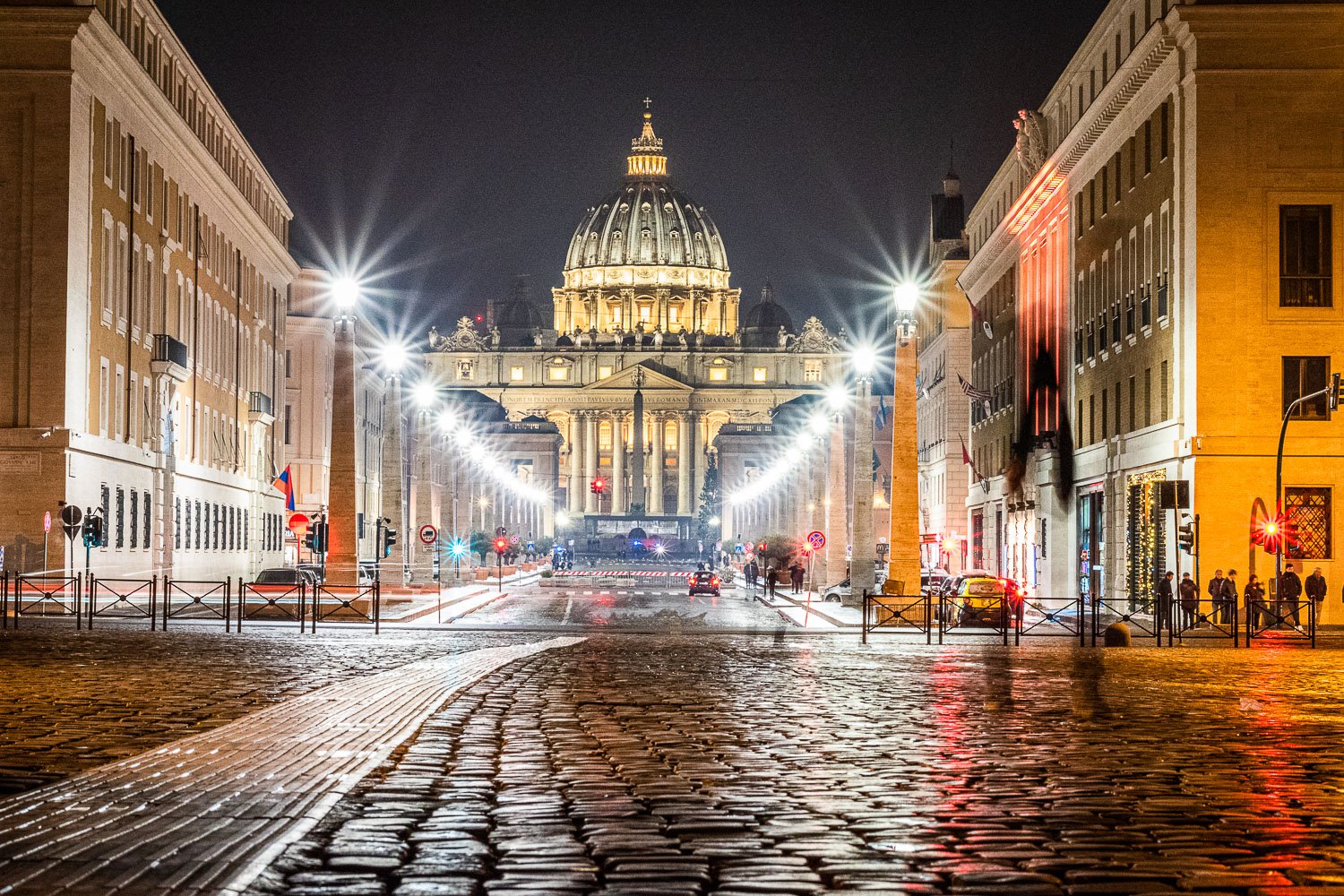In this image, we see a bustling, rain-slicked cobblestone city street at night, illuminated by bright street lights. The road, composed of circular cobblestones arranged in neat rows, glistens from the recent rain. Buildings line both sides of the street, with brown façades featuring numerous windows. Statues and stone pillars topped with lights add to the city's historic ambiance.

In the distance, a grand building with white columns and a large, illuminated dome—perhaps a museum or a significant public building—dominates the scene. The dome, adorned with gold and white lights, peaks with a cross, giving the structure an ancient architectural flair. Scattered cars park along the street, and small groups of people chat on the sidewalks, adding a lively touch to the serene cityscape. The contrast between the bright street activity and the dark night sky enhances the captivating atmosphere of this urban European setting.